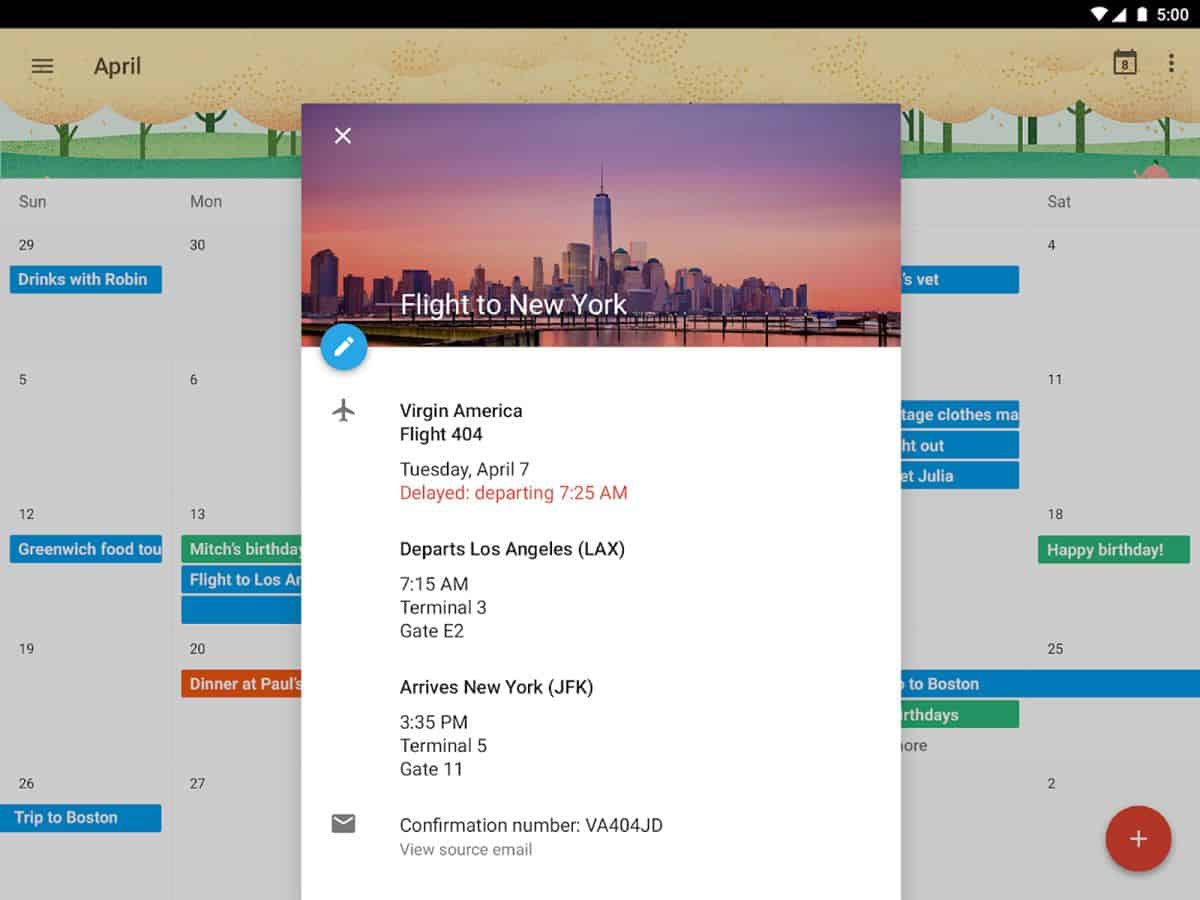In the image, there's a screenshot from a mobile device displaying detailed flight information. At the top right corner, the Wi-Fi signal icon is visible alongside the time, which is showing as 5:00. The battery level is critically low, indicated by a mere 4%. The screenshot details an emergency flight to New York on Virgin America, flight number 404, scheduled for Tuesday, April 7th. The flight, originally delayed, is now set to depart Los Angeles from Terminal 3, Gate E2 at 7:15 AM and will now depart at 7:25 AM instead. The flight is expected to arrive at Terminal 5, Gate 11 in New York's JFK Airport at 3:35 PM. Additionally, the confirmation number for this flight is VA404JD. The mobile interface also includes an option to view a resource email. In the background, there is a calendar displaying schedules and reminders, adding to the context of the travel plans.